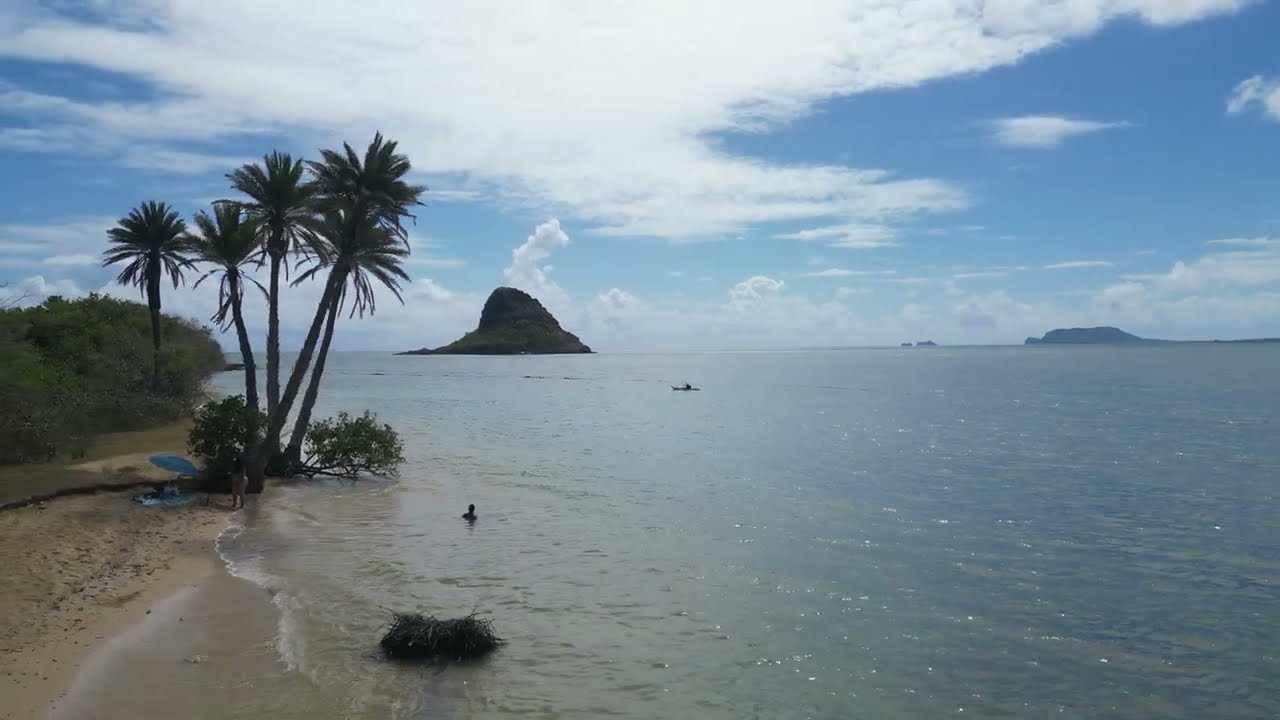This serene, horizontal photograph captures a tranquil tropical beach setting on Oahu, Hawaii, featuring the iconic Chinaman's Hat in the background – a uniquely shaped rock island that resembles a hat. The sky above is a brilliant blue, dotted with delicate cirrus clouds, contributing to the peaceful atmosphere.

In the foreground, a sandy beach stretches from the lower left to the center right of the image, leading to a clear, shallow lagoon or ocean. The shoreline, with its slightly muddy sand, suggests it was taken near the water's edge, possibly where the waves gently lap at the shore. A small rock stands in the shallow water near the beach.

To the left, a charming stand of five palm trees lean slightly toward the center of the image, casting subtle shadows on the sand. Below them, lush green shrubbery thrives, indicating a vibrant, tropical ecosystem. Just behind this grove, the land rises slightly into a hill thick with dense vegetation.

Near the center of the image, a solitary person bathes in the calm waters, adding a human touch to the secluded scene. Further out in the water, a one-person boat navigates either toward or away from the beach, enhancing the sense of adventure and exploration.

On the horizon line, which stretches from the center left to the center right, stands the majestic Chinaman's Hat, a massive rock formation emerging dramatically from the water. Far in the distance on the right, another landmass looms, potentially another island or an isthmus, adding depth to the panorama.

This captivating image evokes a sense of tranquility and natural beauty, perfectly capturing the idyllic essence of a secluded Hawaiian beach.